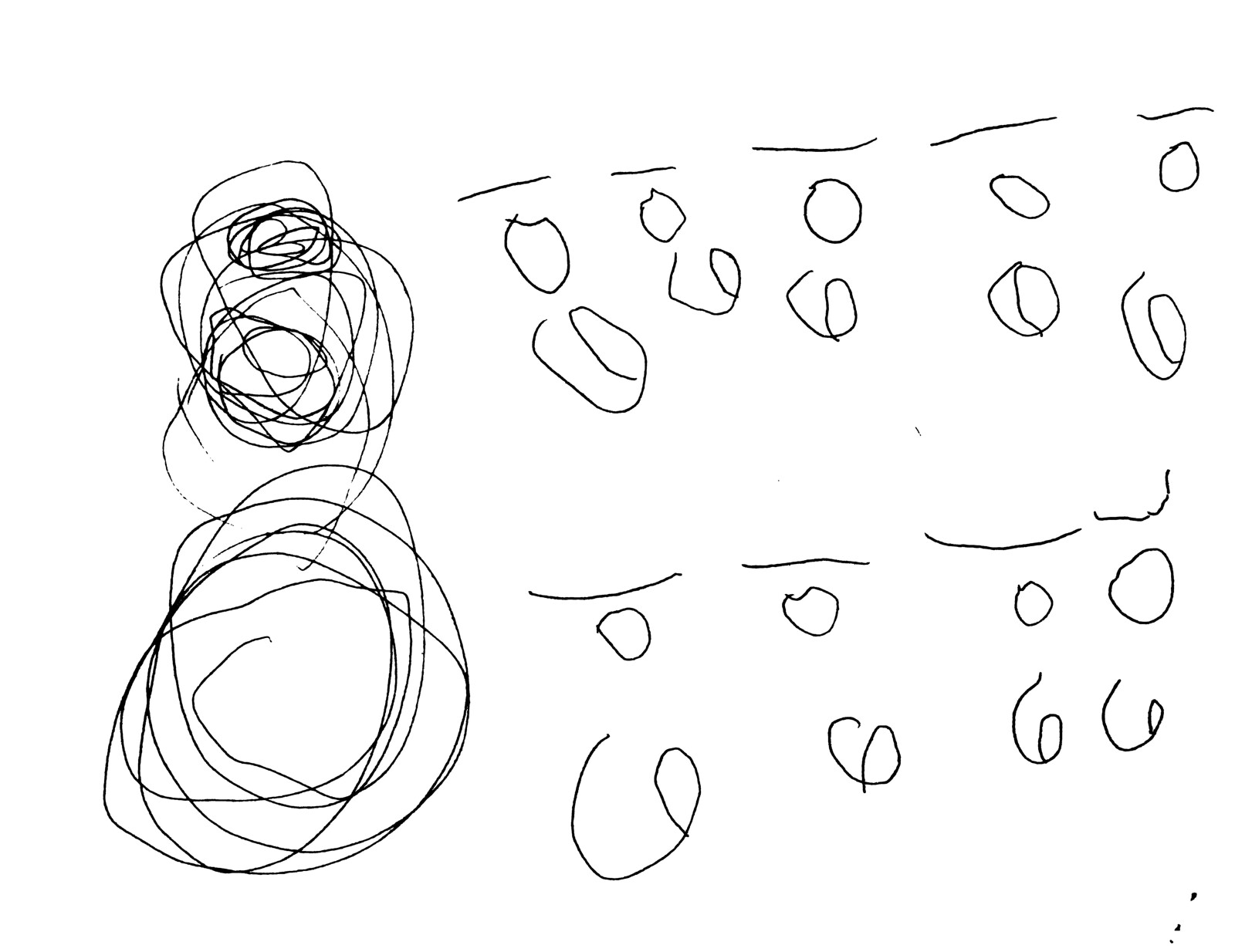The image is a chaotic drawing featuring what appears to be a mix of zeros and sixes, and lines that might represent a rudimentary keyboard layout. The drawing consists of two rows of ten straight lines each, with five lines per row. Below each line in every row, there is a sequence of zeros and sixes: circles (zeros) at the top and sixes below. These, along with the lines, are repeated in a second section underneath the first.

On the left side of the drawing, there are numerous swirling scribbles, possibly indicating that the artist was attempting to get a pen to work by vigorously circling it on the paper. The entire piece seems to have been created with either ink or a very sharp pencil, as the lines are thin yet distinct. The image itself looks as though it may have been photocopied, given the subtle incidental marks on the paper, which do not appear to be part of the main drawing.

The prominent elements—the zeros and sixes—are haphazardly written, suggesting they were done either by a child or by someone with an unsteady hand. The lines, which are slightly angled and not perfectly straight, imply a hurried effort to complete the drawing.